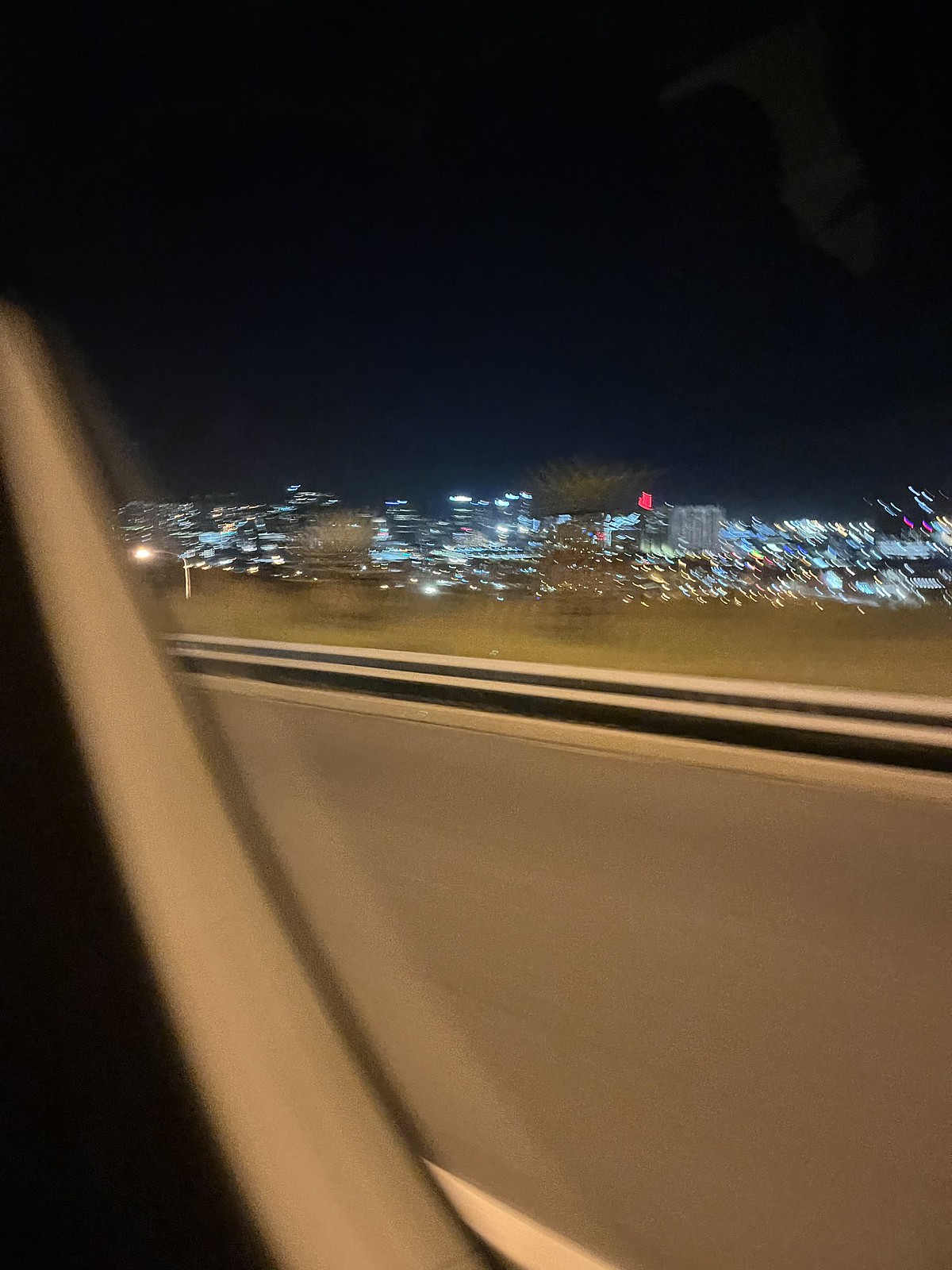A nighttime photograph taken from inside a moving vehicle showcases the contrast between the interior and the outside world. The vehicle's interior features a tannish gray hue, providing a sense of enclosure and comfort. In stark contrast, the world beyond the windshield is a canvas of darkness, with the top half of the image enveloped in a black, starless night sky. As the eye moves downward, the sky transitions into a deep, dark blue near the horizon.

The scene outside is punctuated by a myriad of blurred white lights, horizontally stretched due to the vehicle's motion, creating an effect of speed and movement. Interspersed among these lights are occasional splashes of light blue, adding depth to the night landscape. Towards the foreground, indistinct shapes suggest the presence of trees or bushes, diminishing into brownish tones, offering a hint of nature amidst the man-made illumination.

A curious red speck, square in shape, stands out near the horizon. Its purpose or source is unclear, but it adds an element of intrigue to the otherwise serene night scene.